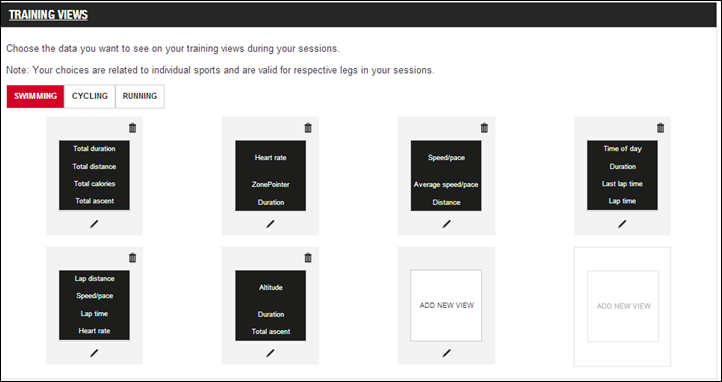The image is a screenshot of a user interface showing options for customizing training data views. At the top of the screen, there's a black bar with the text "Training Views" displayed in white letters. Below this, instructions read: "Choose the data you want to see on your training views during your sessions. Note: Your choices are related to individual sports and are valid for respective legs in your sessions." 

The interface provides customization options for various sports, including swimming, cycling, and running, with swimming currently highlighted in red, indicating it is the sport selected. 

There are several boxes listed with different data metrics available for selection:
1. **First Box**: Total Duration, Total Distance, Total Calories, Total Ascent.
2. **Second Box**: Heart Rate, Zoom Partner, Duration.
3. **Third Box**: Speed, Pace, Average Speed, Pace, Distance.
4. **Fourth Box**: Time of Day, Duration, Last Lap Time, Lap Time, Lap Distance, Speed, Pace, Heart Rate.
5. **Fifth Box**: Altitude (assumed typo in original), Duration, Total Ascent.

Users will choose the appropriate data metrics for each sport, suggesting that the customization will affect the training data display specifically for swimming in this instance.